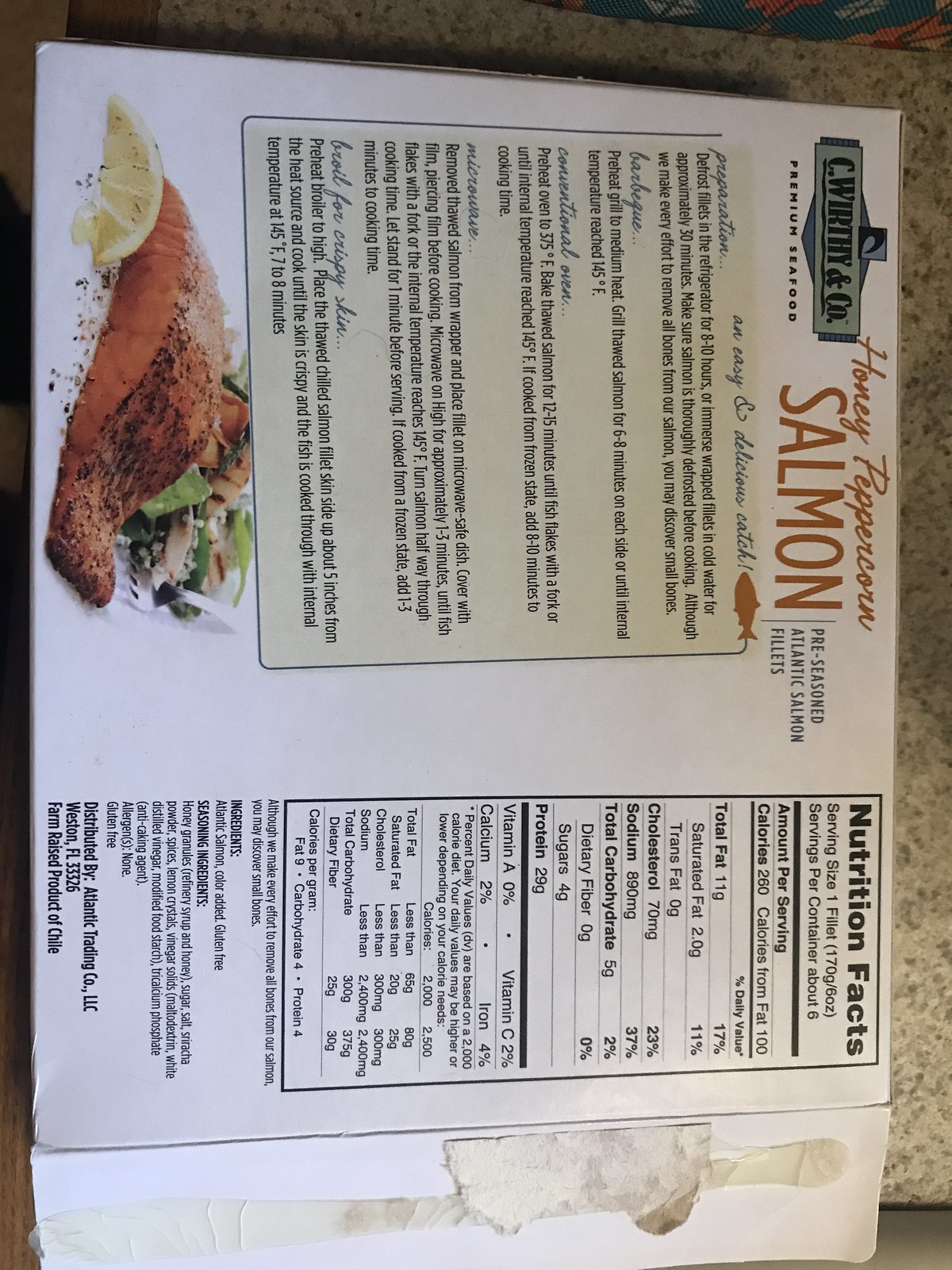The image is a vertical photograph of the back side of a white cardboard packaging for Seaworthy and Company’s premium seafood product, specifically honey peppercorn salmon, showcasing their pre-seasoned Atlantic salmon fillets. The brand's logo is located in the top right-hand corner, clearly identifying the product. Toward the bottom of the image, roughly one third, the nutritional facts are displayed, listing information such as serving size, total fat, cholesterol, sodium, total carbohydrates, protein, vitamins, and minerals. Below the nutritional facts, you can find the ingredient list and distributor details, noting that the product is farm-raised and from Chile, distributed by Atlantic Trading Company, LLC, Western Florida 3326. The left two-thirds of the image feature a detailed recipe and preparation instructions for the salmon fillets, written in black font on an off-white background. Below the preparation instructions, there's an enticing photograph of a prepared salmon fillet garnished with a lemon wedge and accompanied by a fresh salad, emphasizing the product's appeal and serving suggestion.